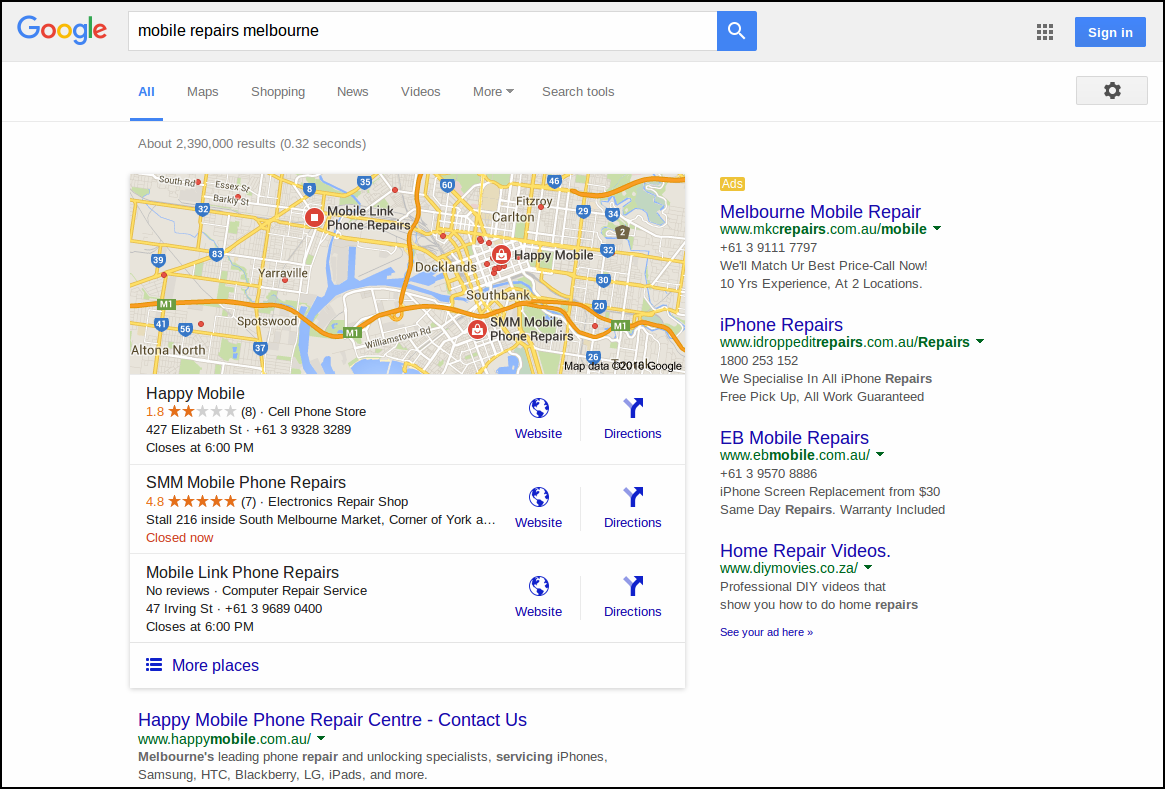The image features a Google search results page for "mobile repairs Melbourne." Prominently displayed is a section on Google Maps, highlighting various mobile repair shops in Melbourne. Below the map, a list of website URLs appears, each linking to different mobile repair service providers. On the right side of the screen, reviews for several of these repair shops are shown. Notable businesses include "Melbourne Mobile Repair," "iPhone Repairs," and "EB Mobile Repairs." Additionally, there are suggested links to home repair videos, offering further assistance for those interested in DIY repair solutions.